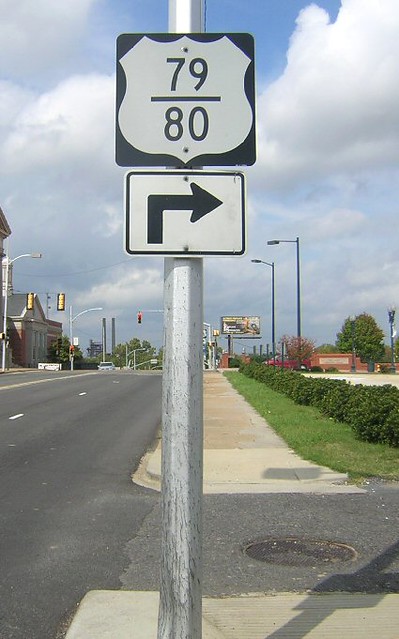This image features a road sign situated in a lightly traveled area, captured in a stretched portrait orientation. The setting is a two-lane road extending away from the photographer's vantage point. The photographer stands on a sidewalk directly in front of the sign, providing a clear view of the details. The sign assembly is mounted on a silver metal post, possibly made of steel or aluminum.

The bottom sign indicates a right turn with a black arrow pointing upward and to the right, set against a white background bordered by a black triangle with rounded corners. Above this directional sign is a U.S. Highway marker displaying an unusual designation: the numbers "79" and "80" separated by a horizontal line, all set within a standard shield-shaped background.

The depiction provides a clear understanding of the road conditions and necessary maneuvers, set in what appears to be a calm and unhurried locale.